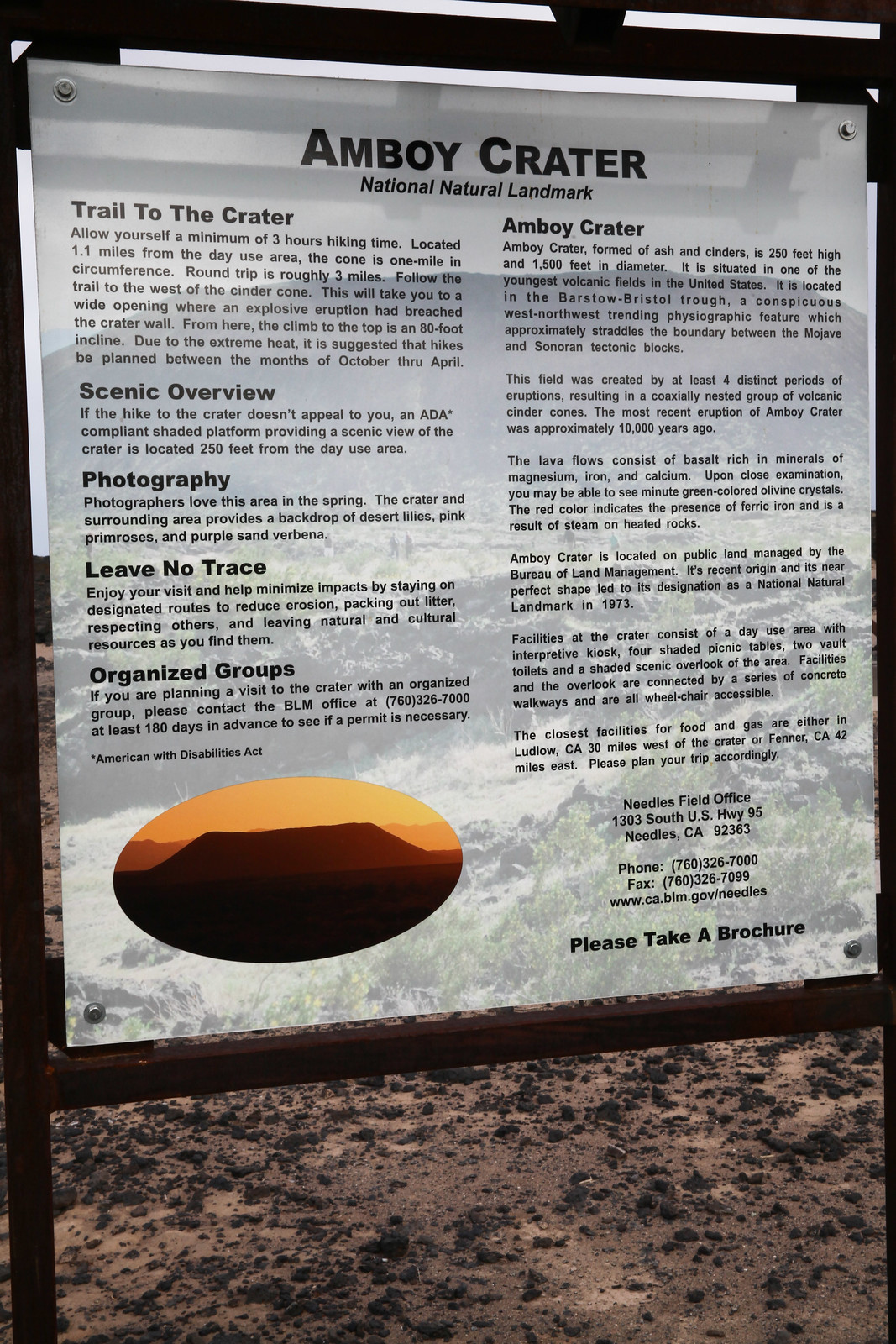The image displays a detailed information sign attached with screws to a black frame, titled "Amboy Crater National Natural Landmark" in bold black letters at the top. The content is divided into two columns of text. The left column contains five sections labeled: "Trail to the Crater," which advises an approximate three-hour hiking time for the 1.1-mile trek, highlighting the breached crater wall and suggesting hikes between October and April due to extreme heat; "Scenic Overview"; "Photography"; "Leave No Trace"; and "Organized Groups," each with descriptive text below. 

The right column features six sections, including another titled "Amboy Crater," with additional information and six compact paragraphs explaining the details. Positioned in the lower-left corner of the sign is an oval photograph capturing the crater at sunset, enhancing the overall visual appeal. Adjacent to this image, contact details for the Needles Field Office are provided: 1303 South US Highway 95, Needles, California 92363, with phone number 760-326-7000, fax number 760-326-7099, and website www.ca.blm.gov/Needles. The sign also includes a prompt at the bottom recommending visitors to "please take a brochure."